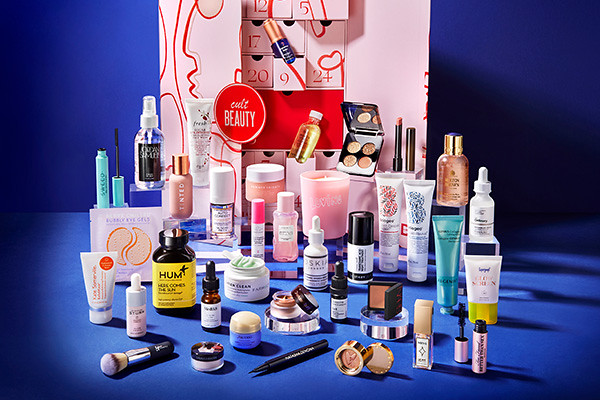This photograph features an intricate display of skincare and makeup products arranged as part of a festive advent calendar collection. The background is a rich bluish-purple hue, enhancing the visual appeal of the products. In the front row, we see a variety of items including a makeup brush, a small lip gloss container, an eyeliner, a foundation bottle, and a mascara. Progressing to the next row, there are slightly larger bottles, such as a lotion bottle, each carefully positioned to create a layered effect.

One particular bottle stands out with the label "Here Comes the Sun," hinting at the overarching skincare theme. The display continues with multiple rows, where the products increase in size as they move toward the back. Some items are elevated on small stands to ensure visibility and prominence. The arrangement culminates with a red circle logo featuring the words "Cult Beauty" in pink font, which sits at the back along with a partially open pink cardboard box, reminiscent of an advent calendar.

Indicating its special theme, this advent calendar display features windows with visible dates such as 12, 5, 17, 29, and 4, suggesting the excitement of discovering new products each day. The majority of the products are in pink or peach tones, adding a cohesive aesthetic, while a few stand out in teal and one in black with a yellow label. This detailed presentation effectively showcases the array of beauty and skincare products included in the Cult Beauty advent calendar, capturing the viewer's attention with its vibrant and festive arrangement.